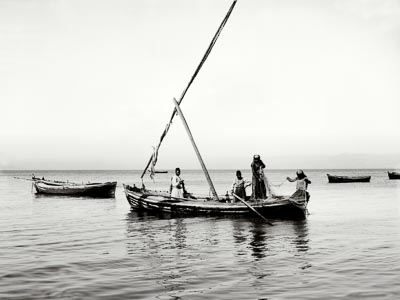In this black and white photo, a central sailboat with four people on board is navigating through a body of water, likely the ocean. The sail appears damaged or collapsed, as evidenced by a twisted mast hanging crookedly. Surrounding the central sailboat are several other canoes or boats, some appearing empty, with the far-right boat mostly cropped out of the frame. The sky is overcast, casting a gray tone over the scene, and waves are visible on the water's surface. One of the four individuals onboard the main boat is wearing a white top. The horizon displays another boat in the distance, adding depth to the photo. It's uncertain whether this image is a vintage photograph or a modern one with a black and white filter.